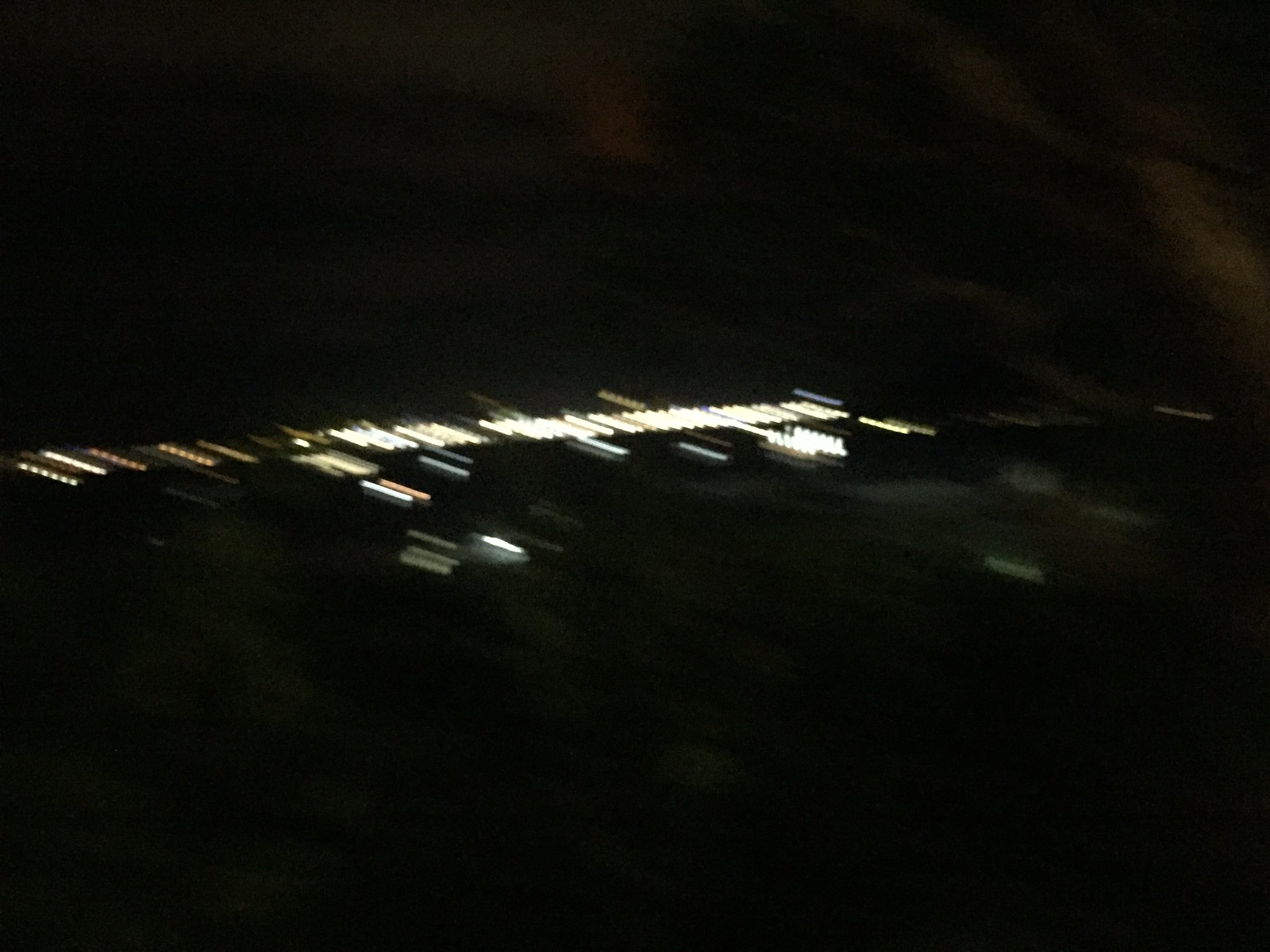This photograph captures a night scene dominated by darkness, with a prominent, slightly blurry strip of light running diagonally from the top left to the bottom right. The light, likely emanating from a distant city, creates an intriguing effect of motion blur, adding a dynamic element to the composition. This faint, stretched light appears to be along the horizon, suggesting an urban landscape far in the distance. The overall impression is that of a long exposure or a 'dragged shutter' shot taken in the dead of night, making the rare light source stand out starkly against the enveloping blackness.